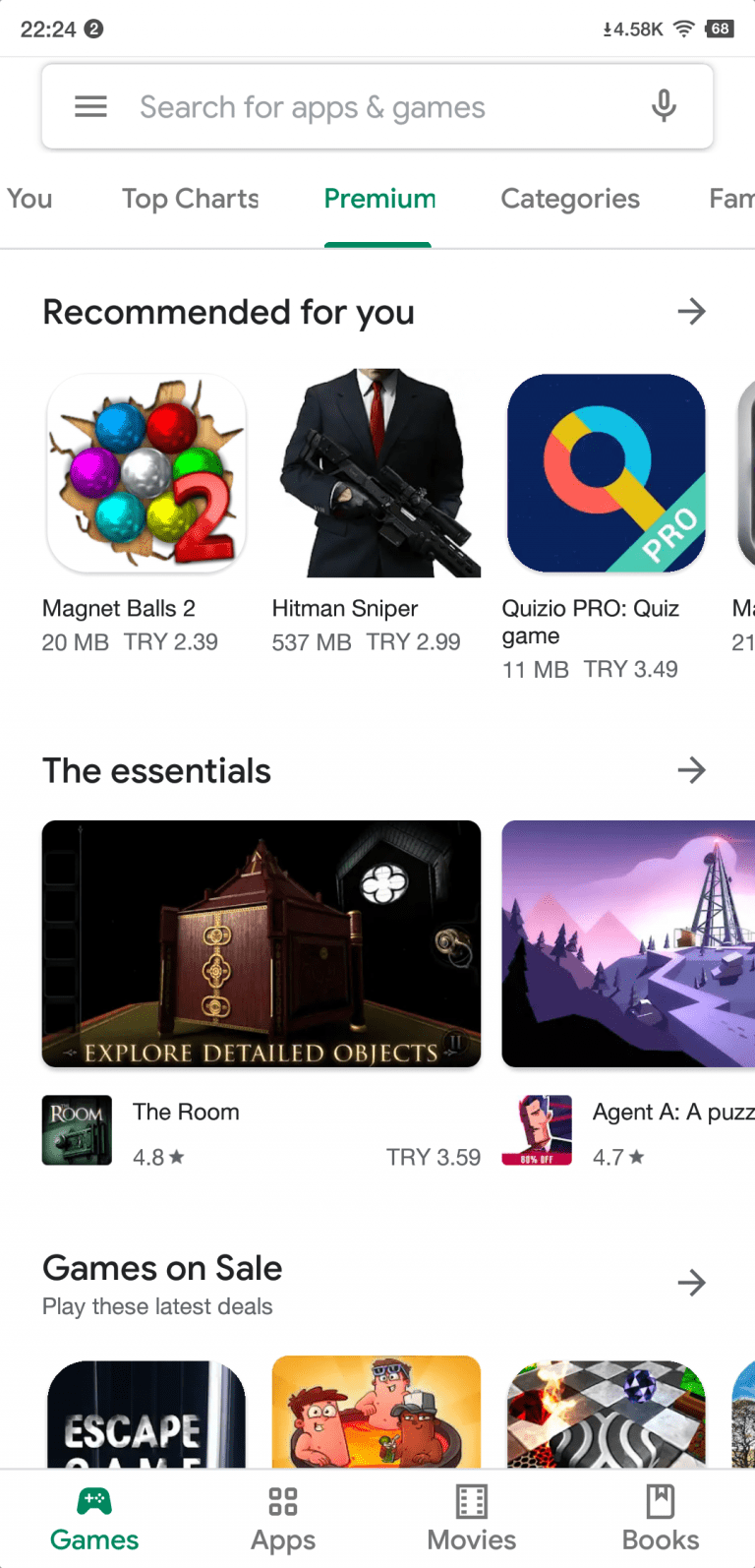The image depicts a screen capture of a mobile phone displaying a landing page for an app store, which is likely the Google Play Store based on its layout and design elements. The top part of the screen includes a status bar, confirming that it is a phone screenshot. 

At the very top, there's a search bar labeled "Search for apps and games." Directly below the search bar are several navigation tabs labeled "For you," "Top charts," "Premium," and "Categories." The section under these tabs is titled "Recommended for you," showcasing several suggested games. The first recommended game is "Magnet Balls," identifiable by its multicolored ball icon. Next is "Hitman Sniper," represented by a character in a suit holding a gun, characteristic of the Hitman series. Another recommendation is "Quiz Pro," with an icon featuring a colorful letter "Q."

Further down, there is a section labeled "The Essentials," which highlights more games such as "The Room" and "Agent A." Below this essential section is an area dedicated to "Games on Sale," indicating more content that users would need to scroll down to view fully. The overall layout and design elements are clear and oriented in a vertical manner, typical of mobile phone displays.